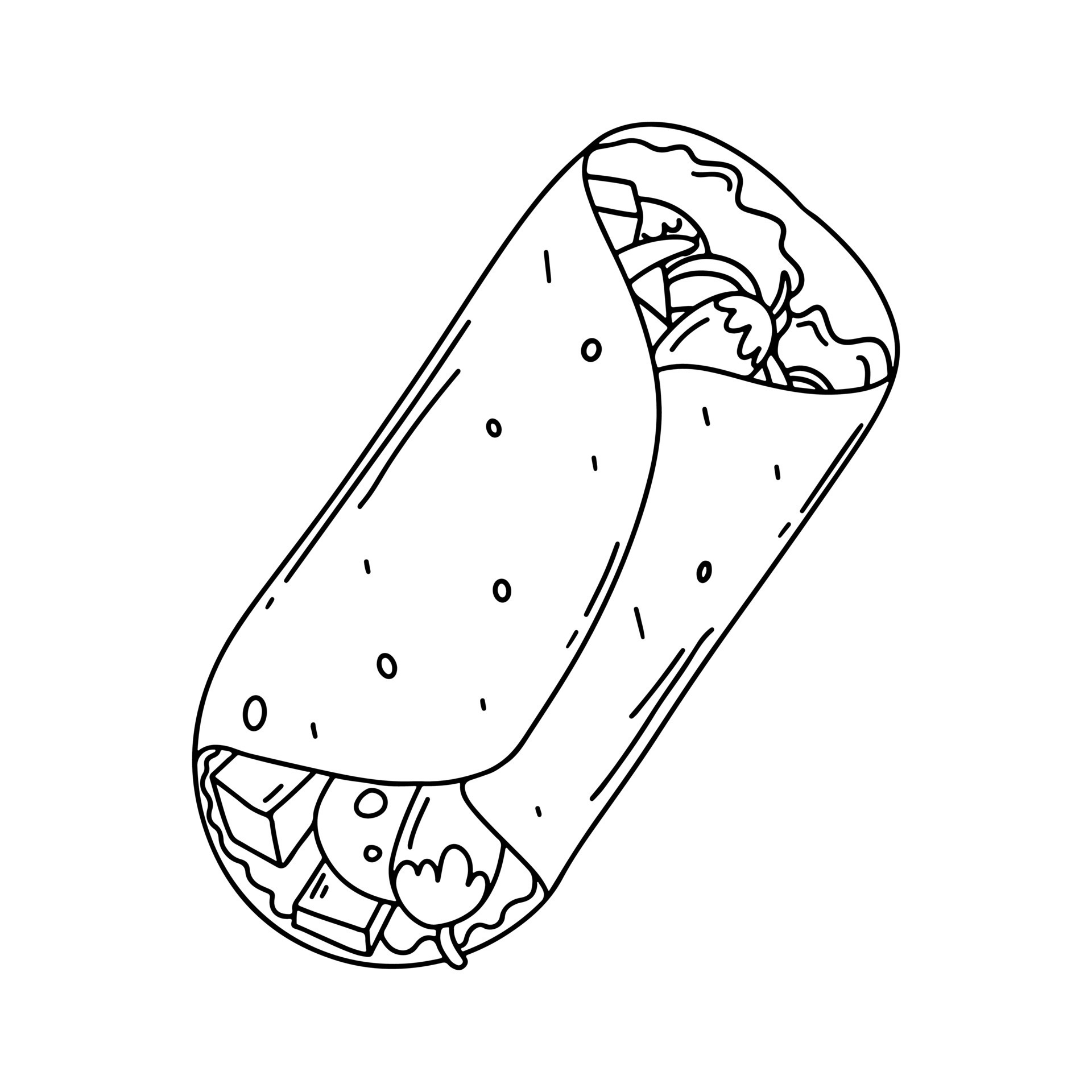This image is a detailed black and white line drawing, likely created with pen. It depicts a folded tortilla or flatbread wrap, rendered at a diagonal angle with one end pointing toward the upper right and the other toward the lower left. The wrap appears hand-drawn and features overlapping folds, with the left side slightly covering the right. The surface of the tortilla is marked with small black circles and vertical lines for texture.

Food items are shown protruding from both ends of the wrap, but their specific identities are ambiguous. Elements resemble cheese cubes or sticks and possibly lettuce, with some participants speculating about the inclusion of pickles or jalapeños. The drawing itself is sparse and restrained, lacking shading or intricate details, and described as not highly artistic. It conveys an impressionistic texture of the tortilla, suggesting a practical yet simple illustration style.